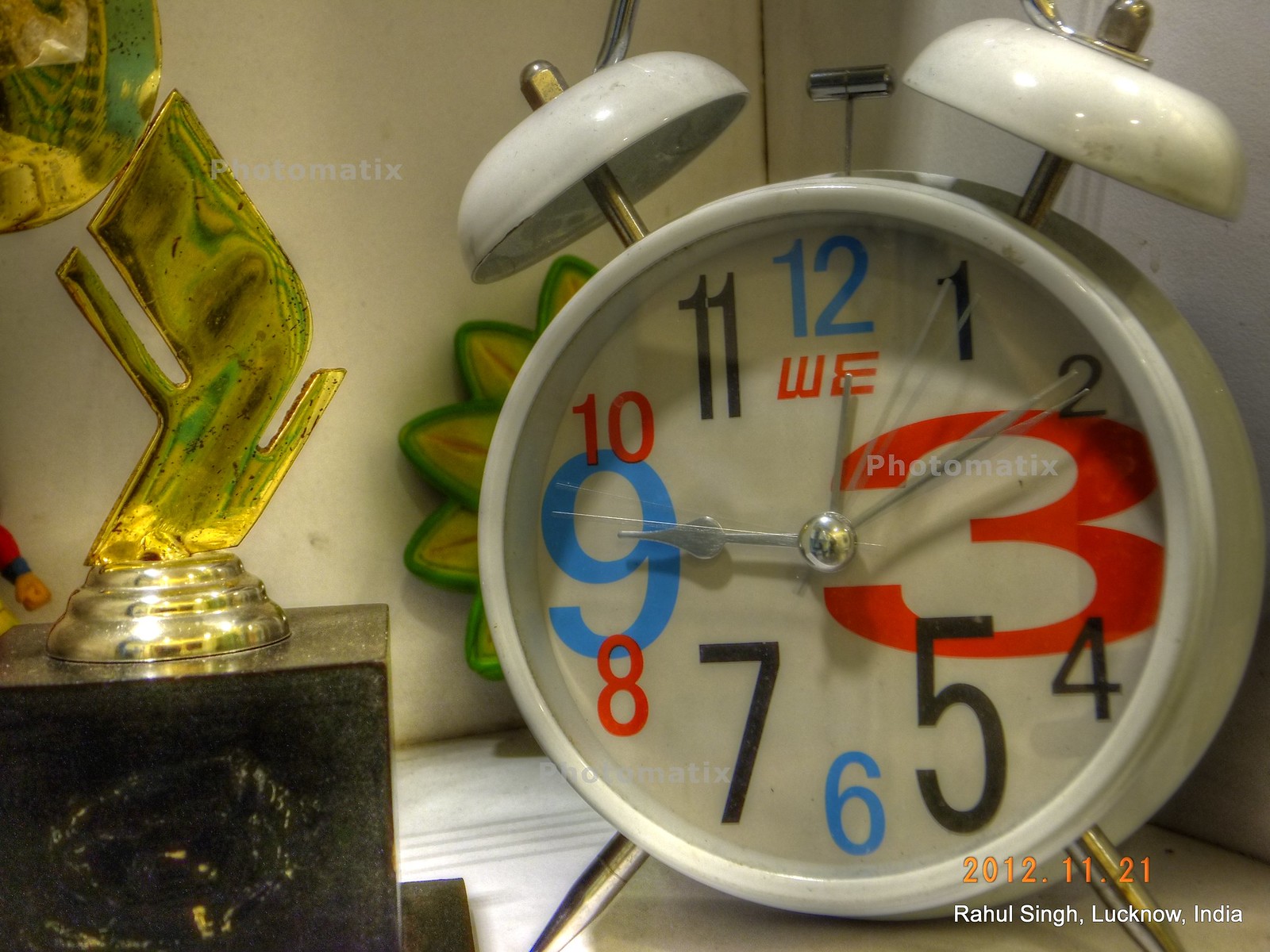The image features a vintage-style alarm clock prominently placed on a dresser. The clock has a circular face with wide, easily readable numerals from 1 to 12, and the time displayed is 12:10. The clock is equipped with two white bells on top, which are activated when the alarm goes off. It rests on a gold stand that adds to its antique aesthetic.

To the left of the clock, there is a trophy, identifiable by its distinct base and golden body that gives it a classic trophy appearance. In the background, a decorative sunflower ornament with green and yellow hues peeks into the frame, adding a touch of whimsy to the setting. The overall scene suggests a cozy, personalized space, likely someone’s bedroom.